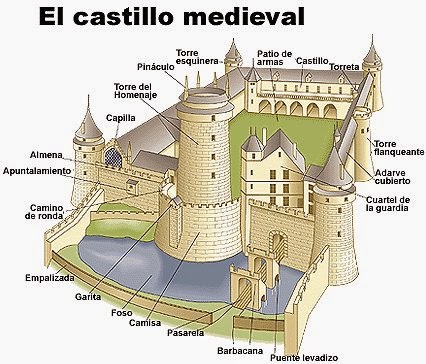This detailed illustration depicts a medieval castle titled "El Castillo Medieval" in bold black letters at the top edge of the image. The castle is meticulously drawn against a light gray background, highlighting its various architectural elements. The front of the castle features a small gate and a drawbridge spanning a blue moat. The castle comprises several smaller buildings within its off-white walls and a tall main tower standing prominently. Four lookout towers are placed strategically at the corners. Inside the walls lies a green, grassy inner courtyard. Around the illustration, black arrows point to different labeled sections in what appears to be Spanish text. Notably, the doorway marked "Capilla" stands out with its bluish hue. The clear and organized layout, complete with a color-coded scheme, enhances the comprehensibility of the castle's structure and components.